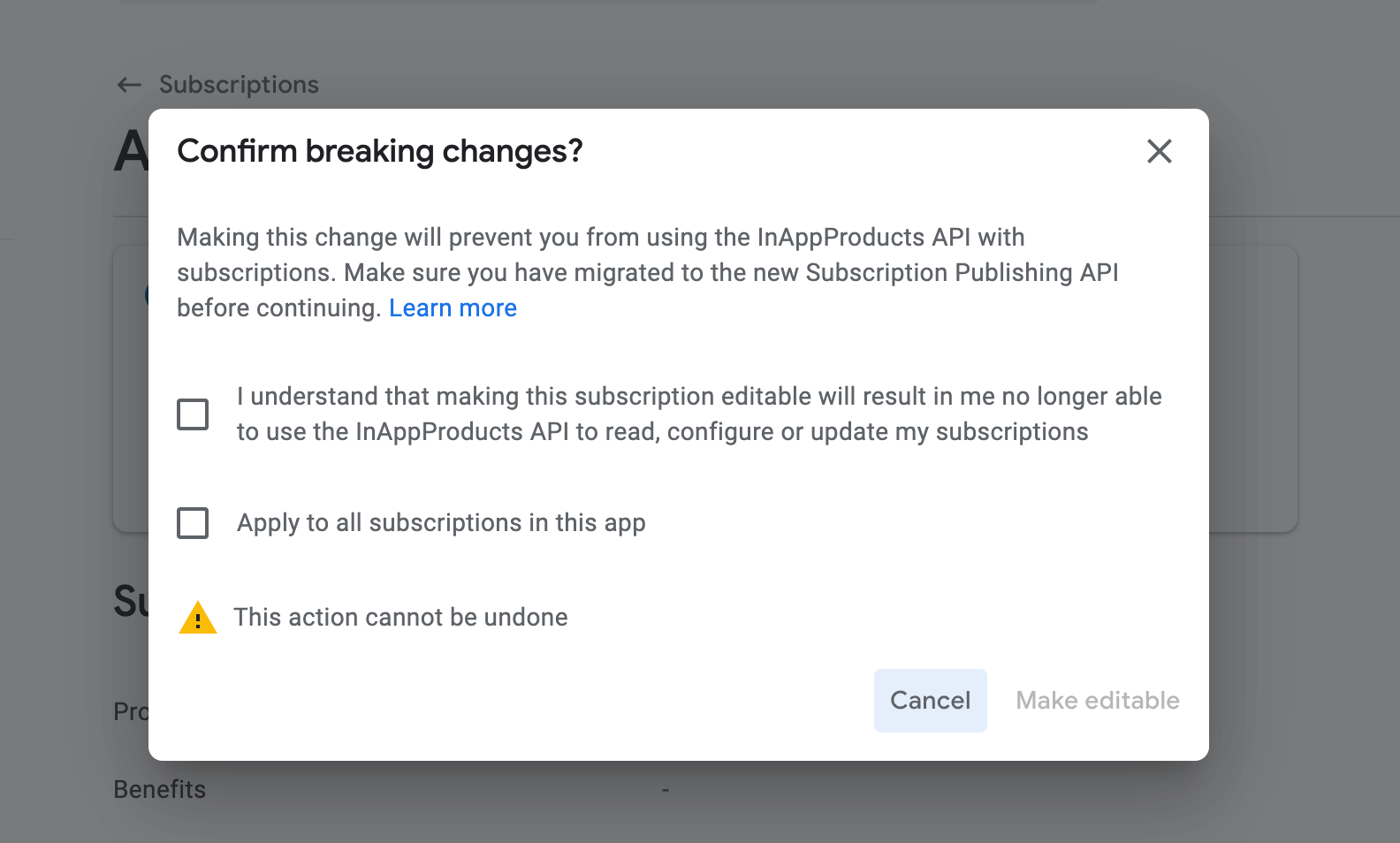The image displays a pop-up dialog box with rounded corners, clearly designed to confirm a critical change. The heading of the pop-up, written in black font, reads "Confirm Breaking Changes?". Below this heading, a warning message is provided in a smaller, light gray font: "Making this change will prevent you from using the in-app products API with subscriptions. Make sure you have migrated to the new Subscriptions Publishing API before continuing. Learn more." The "Learn more" text is blue, indicating that it is a clickable link.

There is an unchecked tick box accompanied by a warning in smaller dark gray or black font: "I understand that making this subscription editable will result in me no longer being able to use the in-app products API to read, configure, or update my subscriptions." Another tick box follows with the option, "Apply to all subscriptions in this app", indicated to its right.

A yellow cautionary triangle with a black exclamation mark inside signals a critical warning: "This action cannot be undone."

At the bottom right of the dialog, there are two buttons with rounded edges. The first is a light gray button labeled "Cancel" in black font. Adjacent to it is a disabled "Make Editable" button, also in light gray to indicate that it is not clickable.

In the background, at the top left, "Subscriptions" is written in black font next to a left-pointing arrow. Just below, part of a bold capital "A" is visible.